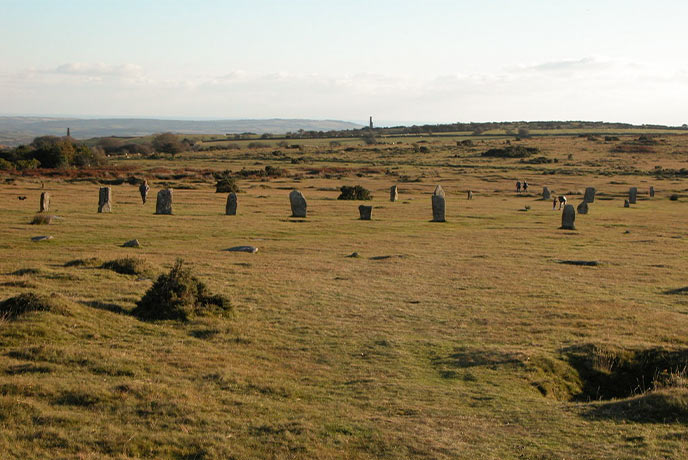This photograph showcases an expansive open field with a mix of green and brown grass, suggesting sun-scorched patches. Scattered throughout the field are numerous ancient stone tombstones of varying shapes and sizes—some rectangular, spherical, and pyramid-like. Notably, there are fewer stones closer to the camera, but they become more prevalent towards the middle of the scene. On the far left, a child can be seen running between two stones. Further to the right, two people stand close together, and nearby, another child with an adult bending down are nestled among three stones and a smaller one adjacent to them. The background features a small tree line and a few distant stones, beyond which lies another clearing with gentle rolling hills. There is sparse shrubbery towards the back hill, with some also near the camera on the left. The sky above is gray with faint outlines of clouds, adding to the serene yet somber atmosphere of what appears to be a very old, open graveyard on a plain.